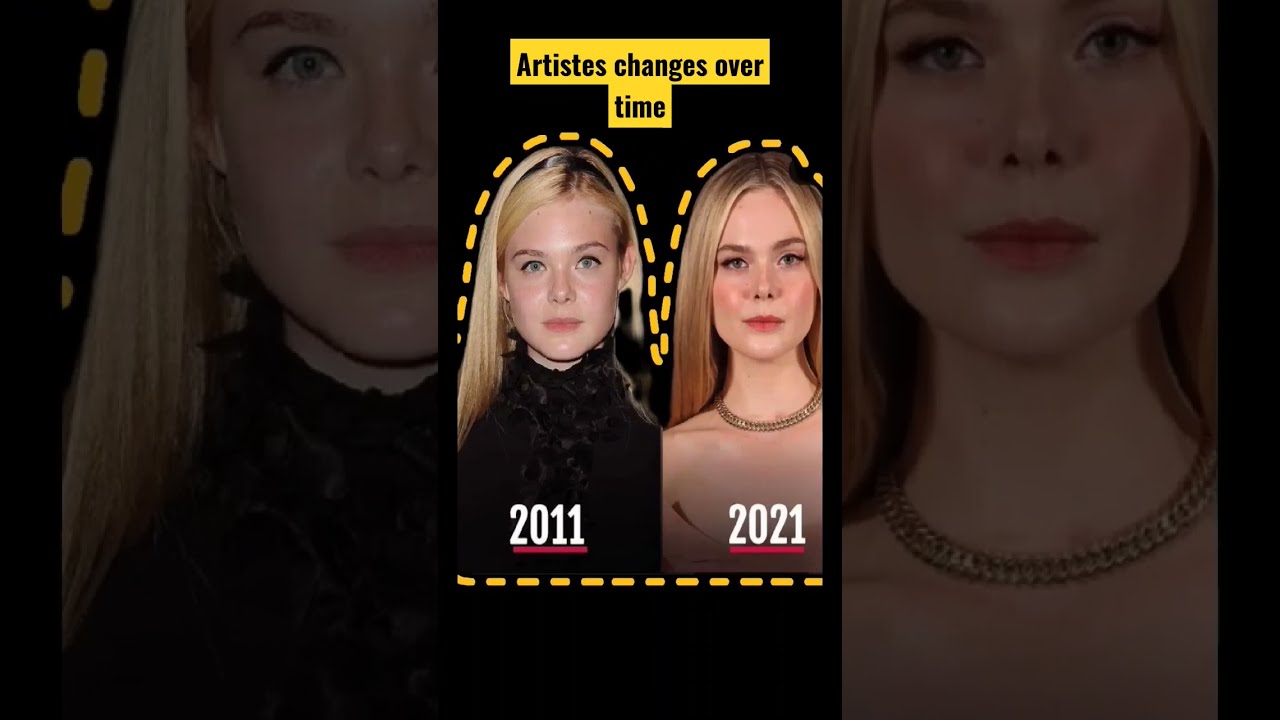The image is a screen grab of a vertical video displayed on a landscape screen, surrounded by a echoed background to fill up the entire frame. At the top, black font on a yellow background reads "Artistes Change Over Time." The main focus is on two photos of Elle Fanning, the actress and sister of Dakota Fanning, comparing her appearance from 2011 and 2021. The 2011 version of Elle, on the left, shows her looking younger with sparser eyebrows, blonder hair, and a dark, more covered outfit. The 2021 version, on the right, displays her with noticeable makeup, fuller lips, and hair that fades from natural blonde to a red or pink hue at the tips. She appears to be wearing fewer clothes, adorned with a chunky necklace and a strapless pink dress. Both images have a segmented yellow outline around them, with the years "2011" and "2021" in white text, underlined in red below each respective photo. This visual comparison highlights Elle Fanning's evolution over a decade.